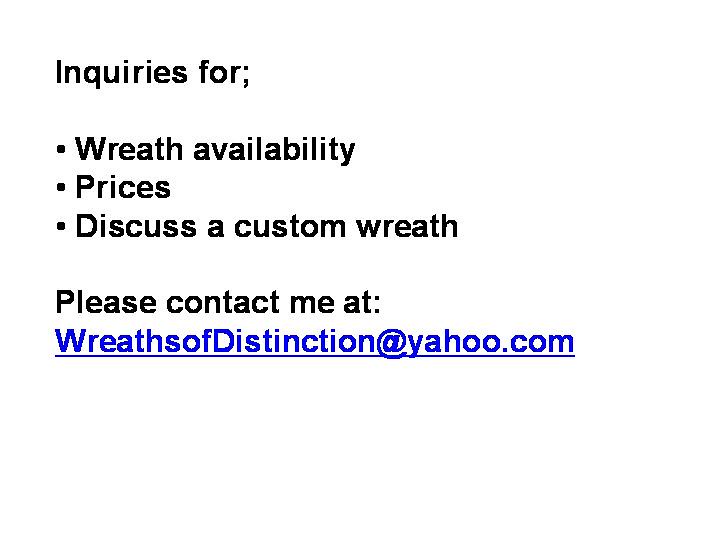The image displays an advertisement or a request, formatted similarly to an email, with a predominantly white background and a mix of black and blue text. The top of the image in black text reads "Inquiries for" followed by a semicolon, and is accentuated by three black bullet points. These points detail the services offered: "Wreath Availability," "Prices," and "Discuss a Custom Wreath." Below these points, further directions are provided in black text: "Please contact me at," followed by an underlined blue email address, "wreathsofdistinction@yahoo.com." The email is prominently placed on the white background, emphasizing its importance for potential customers looking for customized wreaths, possibly for holidays, funerals, or various events. All text appears aligned to the left side of the image, maintaining a clean and straightforward design.